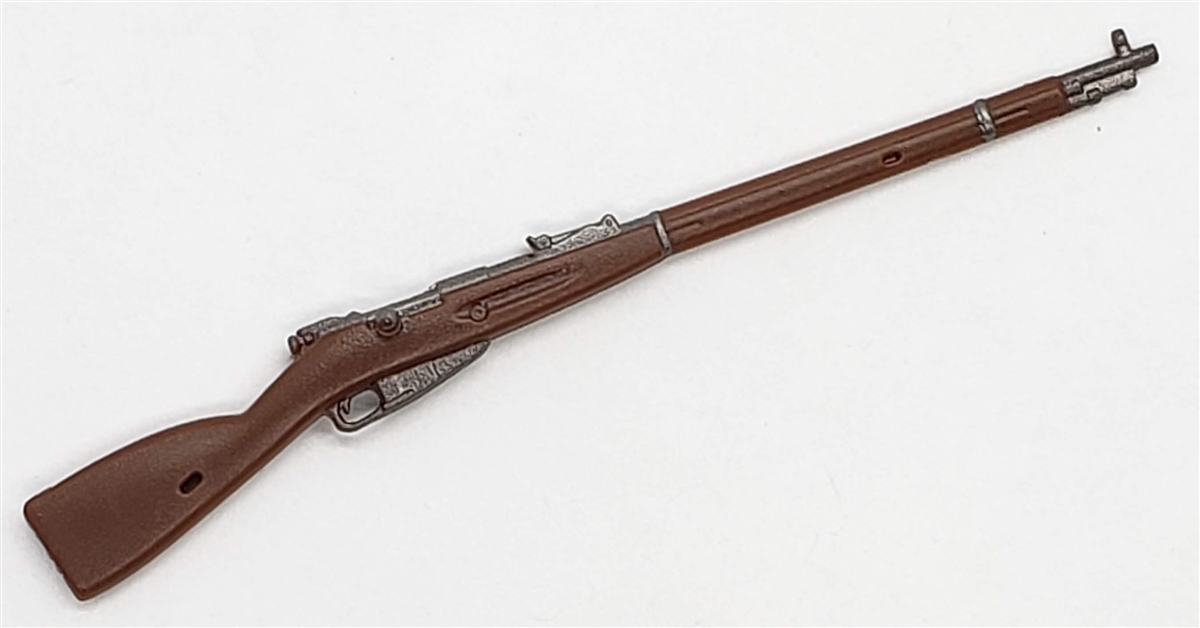The photograph is of a rifle that appears to be a detailed replica or model rather than a functioning firearm. The barrel, painted black, is pointed towards the top right corner, while the buttstock, crafted to resemble brown wood, is angled towards the bottom left corner. The gun is detailed with a black-painted section where the ejection port and sights are typically found, along with a black trigger, trigger guard, and magazine holder. The overall shape, reminiscent of old war rifles possibly from World War I or World War II, features a bolt action mechanism indicated by a metallic bolt mid-gun. The intricate model, with affixed parts, suggests a non-functional design, as the components which would normally be removable are seamlessly melded into the structure. The rifle rests on a flat, light gray surface within a rectangular frame, where the length of the top and bottom sides is twice that of the left and right sides. Despite its metallic appearance, the spots where oxidation might occur are also artistically represented, enhancing the lifelike qualities of the model.